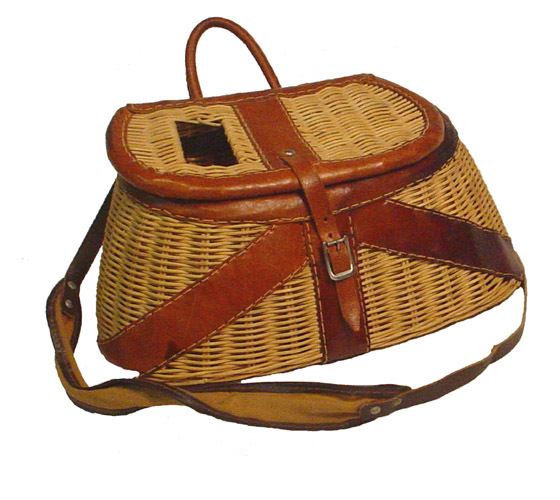This image features an antique, rattan handbag set against a pure white background. The handbag, crafted from light tan woven rattan, showcases an oval-shaped base that tapers toward the top, giving it a distinctive basket-style appearance. Both the body and the oval lid are adorned with dark brown leather accents, particularly along the edges. A prominent feature is the leather strap that secures the lid to the main body, alongside a leather handle at the back and a secondary shoulder strap. The object is positioned diagonally in the center of the image, allowing clear views of the front, side, and top. This detailed presentation, with additional colors in the scene being dark brown, black, silver, and light brown, suggests the handbag's age, indicating it could be an antique, possibly 50 to 100 years old. The photograph's clean, isolated setting implies it could be an advertisement, likely for a site selling vintage or fashion items.